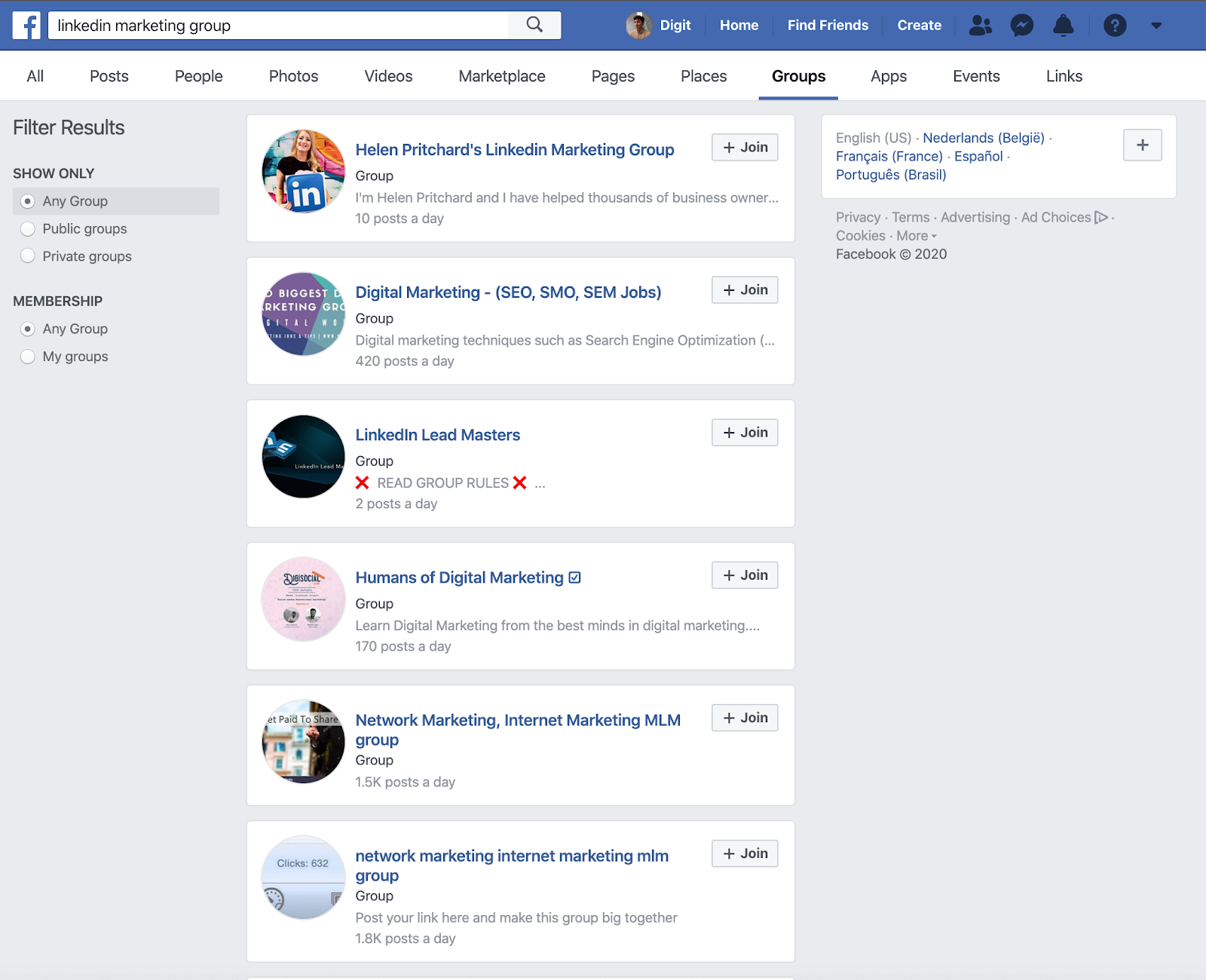The image depicts what appears to be an interface merging elements of Facebook and LinkedIn. At the top of the screen, there is a blue bar spanning from the left to the right. On the left side of this bar is an 'F' symbol, indicative of Facebook's branding. Next to this, towards the right, is a search bar. To the right of the search bar, there is a numerical digit and a small profile picture.

Further to the right on the blue bar are navigation options labeled 'Home,' 'Find Friends,' and 'Create,' followed by a set of four icons and a drop-down menu next to a question mark.

Below this bar, an options menu extends horizontally across the interface, offering categories such as 'All Posts,' 'People,' 'Photos,' 'Videos,' 'Marketplace,' 'Pages,' and 'Place.' Currently, the 'Groups' section is open, displaying various joinable groups.

Here, six groups are listed with brief descriptions and the option to join by clicking a plus symbol. The first group is "Helen Pritchard's LinkedIn Marketing Group," accompanied by a description and their post count. Following this are additional groups: "Digital Marketing," "LinkedIn Leadmasters," "Humans of Digital Marketing," "Network Marketing One," and "Network Marketing Internet Marketing Group."

To the left of the groups, there is a gray sidebar titled 'Filter Results.' It features options to narrow down the group listings by 'Show Only,' with filters like 'Any Group,' 'Public Groups,' and 'Private Groups.' Another filter, 'Membership,' allows users to toggle between 'Any Group' and 'My Groups.'

On the right side of the filter, there is a language selection option, allowing users to switch from English to other languages such as French and Spanish. At the bottom of the interface, standard copyright information is displayed.